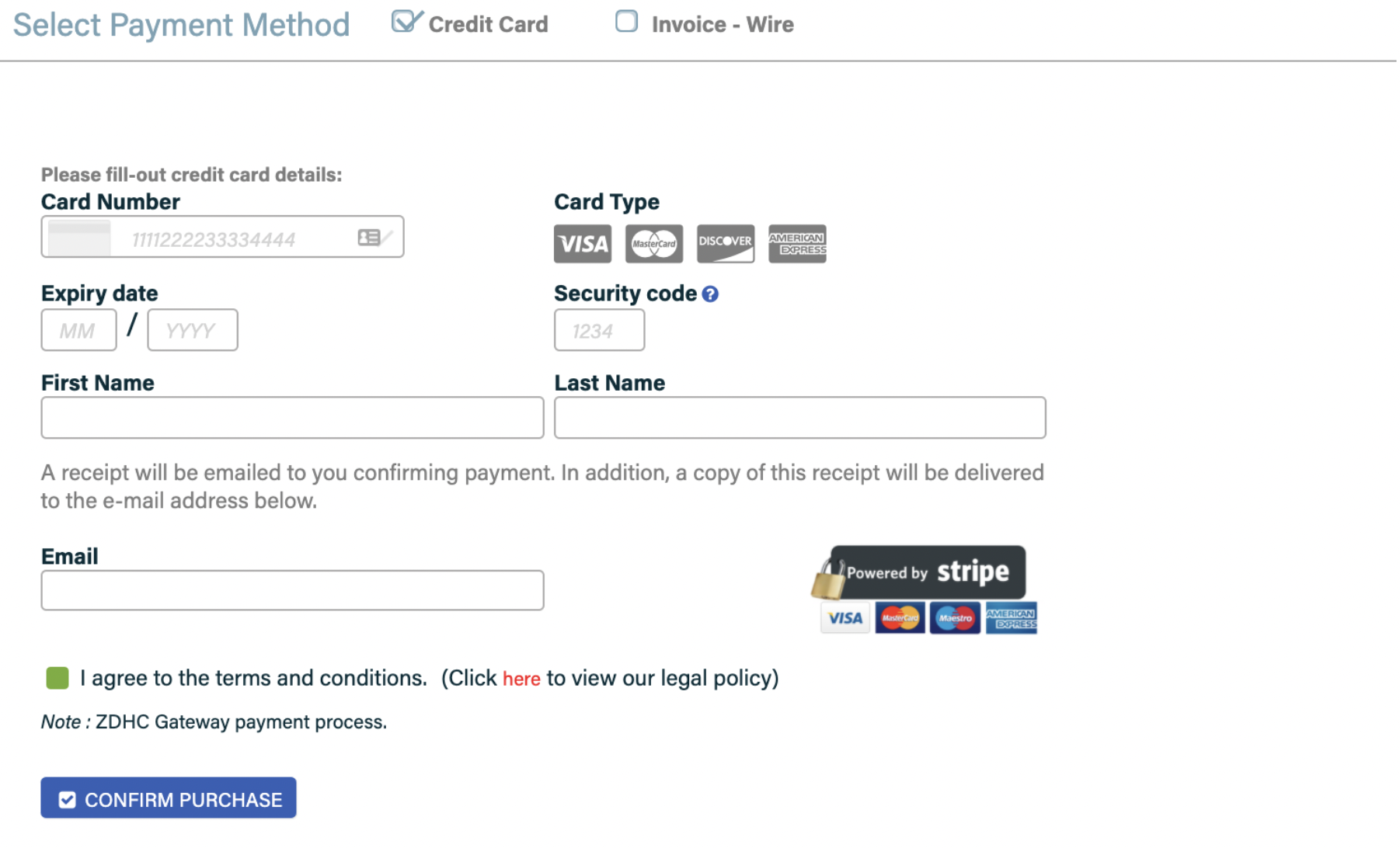The image displays a section of a website's checkout page, specifically tailored for selecting a payment method. At the top left, the text "Select Payment Method" is prominently displayed in light blue. Adjacent to this, a light blue squared box contains a blue check mark, indicating the selection of the payment method. To the right of this box, the words "Credit Card" are printed in black text. Further right, after a small empty space, there is another small blue box followed by the text "Invoice/Wire" in light black.

Below this segment, there are several input fields for entering payment details. On the middle left, a box is labeled with the instruction "Please fill out credit card details." Directly underneath, the label "Card Number," bolded and in a dark blue text, precedes a text box filled with a placeholder card number: "1111-222-3333-444."

Further down, the label "Expiry Date" (also bolded and in dark blue text) is situated above two smaller boxes, which are placeholders for the month (MM) and year (YYYY) of the card’s expiration. Below these fields, there are two more boxes for entering personal information—one labeled "First Name" and the other "Last Name," both of which are currently empty.

At the very bottom left of the image, there is a small blue box with the text "Confirm Purchase," indicating the button for completing the transaction.

The design uses a consistent light blue color for guidance text and darker blue for important labels, providing a clear and user-friendly interface for the checkout process.